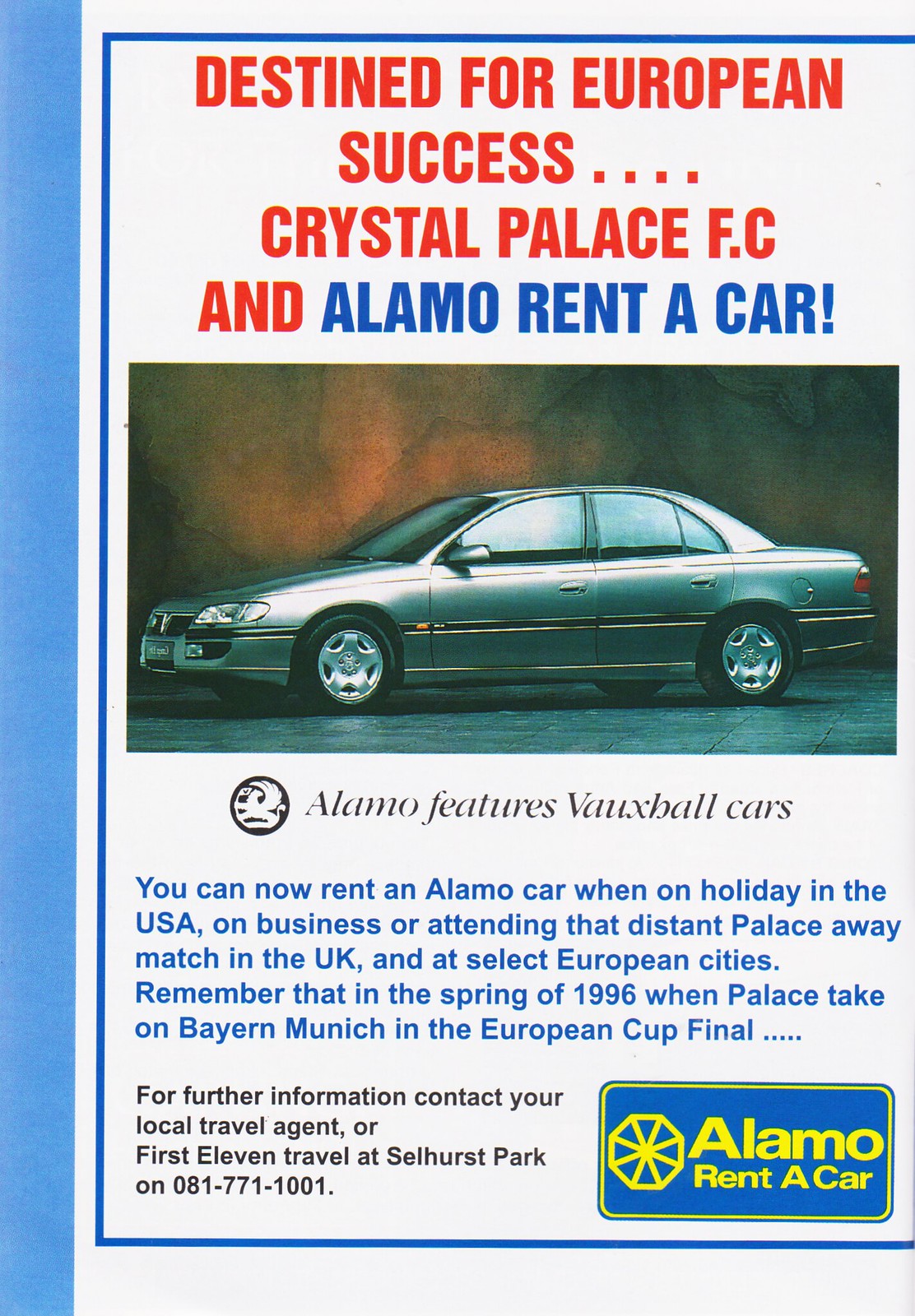This advertisement, possibly from a magazine, features a sleek design with a white background complemented by a blue vertical border running down the left side, along with a thinner blue border outlining the top, left, and bottom sides. The top of the page prominently displays in bold red capital letters, "Destined for European Success…. Crystal Palace F.C." Below this, in blue text, it reads "Alamo Rent-A-Car!"

Central to the advertisement is an image of a gray sedan oriented to the left. Beneath the vehicle, in black italicized text, it states, "Alamo Features Vauxhall Cars." Following this, in smaller blue text, it details, "You can now rent an Alamo car when on holiday in the USA, on business, or attending that distant Palace away match in the UK, and at select European cities. Remember that in the spring of 1996, when Palace takes on Bayern Munich in the European Cup Final…."

At the bottom of the page, further instructions are given in black text: "For further information, contact your local travel agent or First 11 Travel at Selhurst Park on 081 771-1001." The poster concludes with the Alamo Rent-A-Car logo in the bottom right corner, featuring a blue background and yellow text, "Alamo Rent-A-Car," next to an emblem.